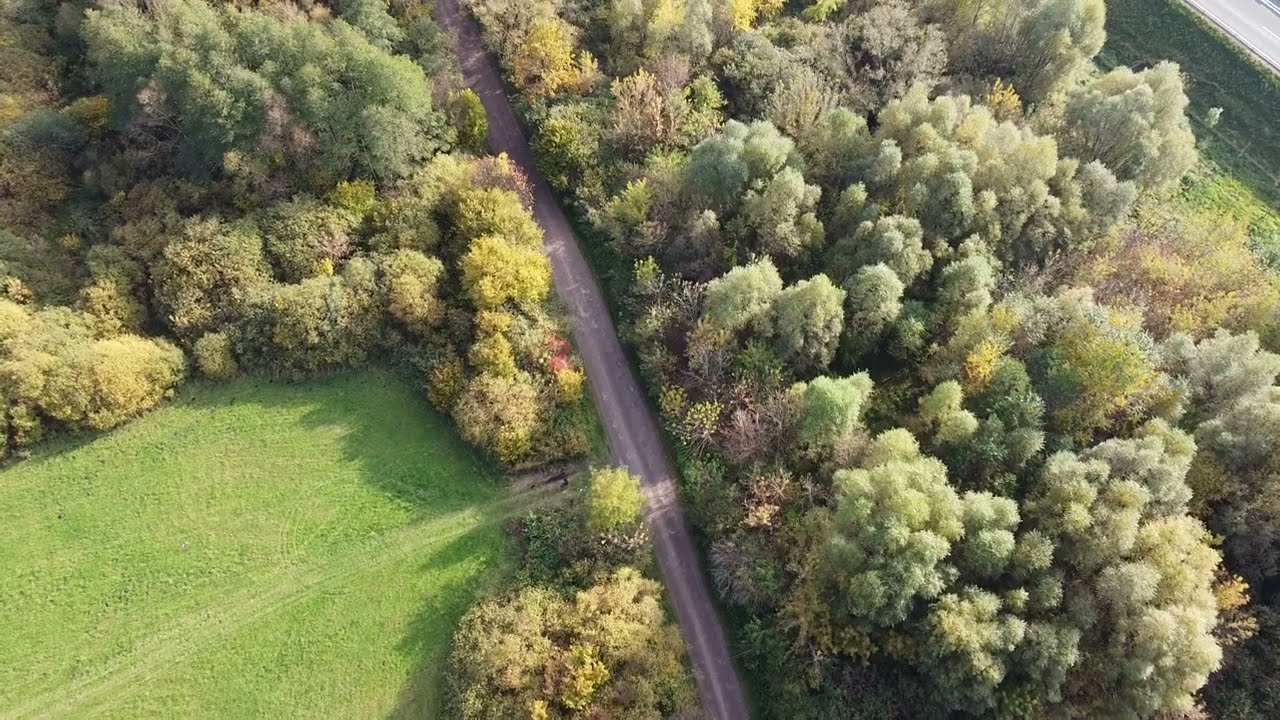This detailed aerial view captures a winding road that starts from the bottom center and meanders towards the top left, surrounded by lush greenery. The road is an unmarked, light-gray pavement, suggesting a rural or less-traveled path. On both sides, the landscape is rich with trees of varying heights and shades of green, forming dense, vibrant foliage. In the bottom left corner, a large, mowed field of vivid green grass is distinctly visible, encircled by trees, with evidence of a frequently-used trail or path leading into the road. On the right side of the image, the greenery continues thickly, except for the upper right corner where another road—a traditional blacktop—appears, offering a contrast to the central unmarked road. The setting is clearly daytime, providing excellent visibility of the diverse foliage and the serpentine path cutting through this verdant landscape.